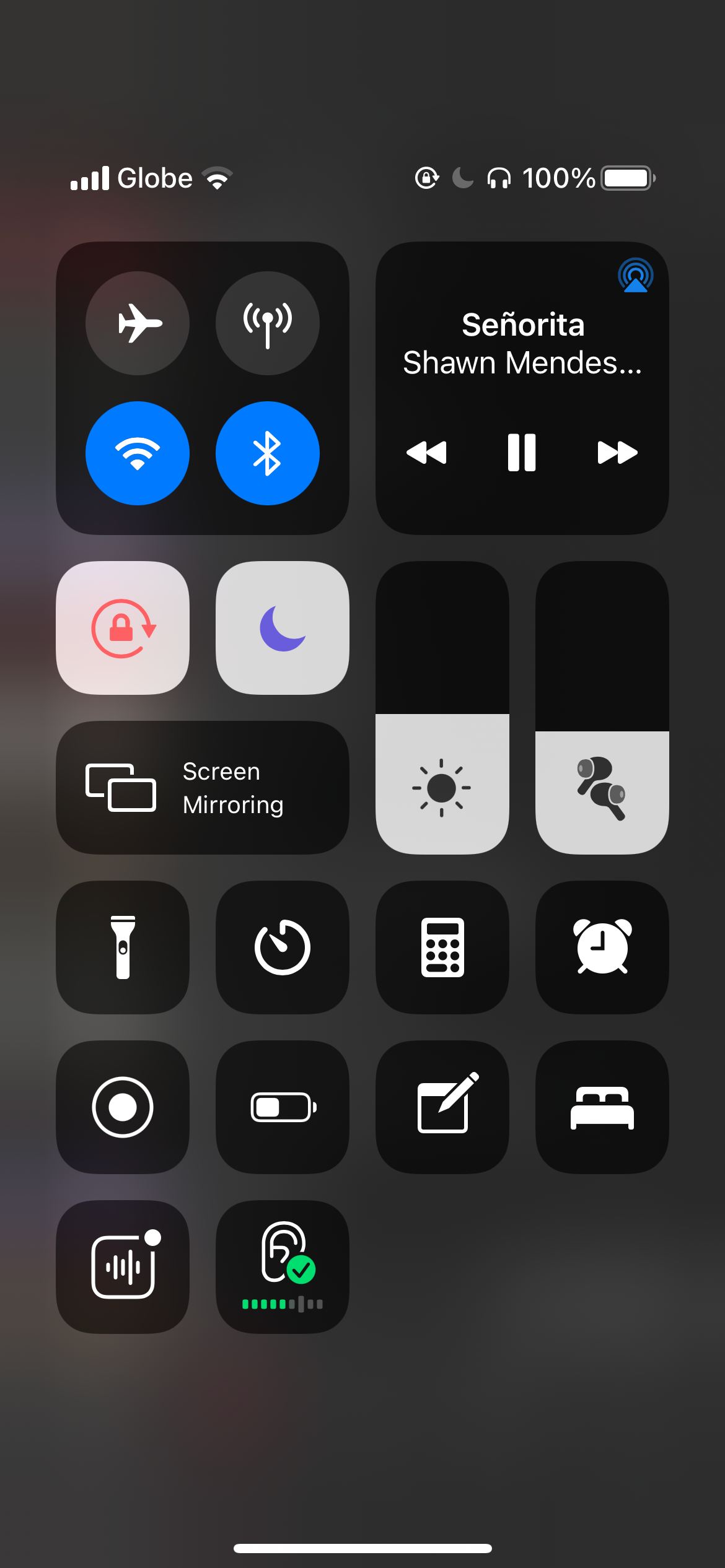The image appears to be a screenshot of a smartphone interface displaying various status icons and control symbols in a well-organized layout. 

In the top section, the status bar shows a full-strength data signal with five bars labeled "GLOBE" and a Wi-Fi signal with three out of four bars. Adjacent to these, there is a gray lock icon encircled by an arrow, which is partially obscure and hard to identify. A gray crescent moon icon, likely indicating do-not-disturb mode, and a headphone icon are also present. The battery status is depicted as fully charged at 100%, represented by a white battery icon rimmed in gray.

Below this, the screen splits into two black squares containing various icons. The square on the left displays four circles. The top-left circle shows a white airplane icon signifying airplane mode, while the top-right circle features a white wireless signal symbol, both set against gray backgrounds. The bottom-left circle displays a white Wi-Fi icon on a blue background, and the bottom-right circle shows a Bluetooth symbol indicating active Bluetooth audio.

The square on the right features a blue triangle or pyramid shape with three outlined circles at the top right corner. Below, the text "Senorita Shawn Mendes..." is visible, accompanied by media control icons: rewind, pause, and fast-forward. Below this media control section, there are two smaller white squares with icons. The left square shows a red padlock encircled by an arrow, and the right square displays a blue crescent moon icon. 

Underneath, "Screen Mirroring" is labeled on a black background with two outlined black squares nearby. To their right, there are two rectangles; the top one is black with a gray sun icon, and the bottom is white with two AirPods icons. Below these are rows of additional control icons, each set in black squares. The icons include:
1. Flashlight
2. A gauge with a left-pointing notch
3. Calculator
4. Clock
5. Record symbol (circle with a dot)
6. Battery icon (half full)
7. Notepad and pencil
8. Bed icon
9. Sound waves with a small circle
10. Two arrows forming a circle with a green check mark.

Each symbol is intricately designed and clearly represents various functions and statuses of the smartphone. The overall design of this interface is detailed and function-oriented, providing quick access to essential features.